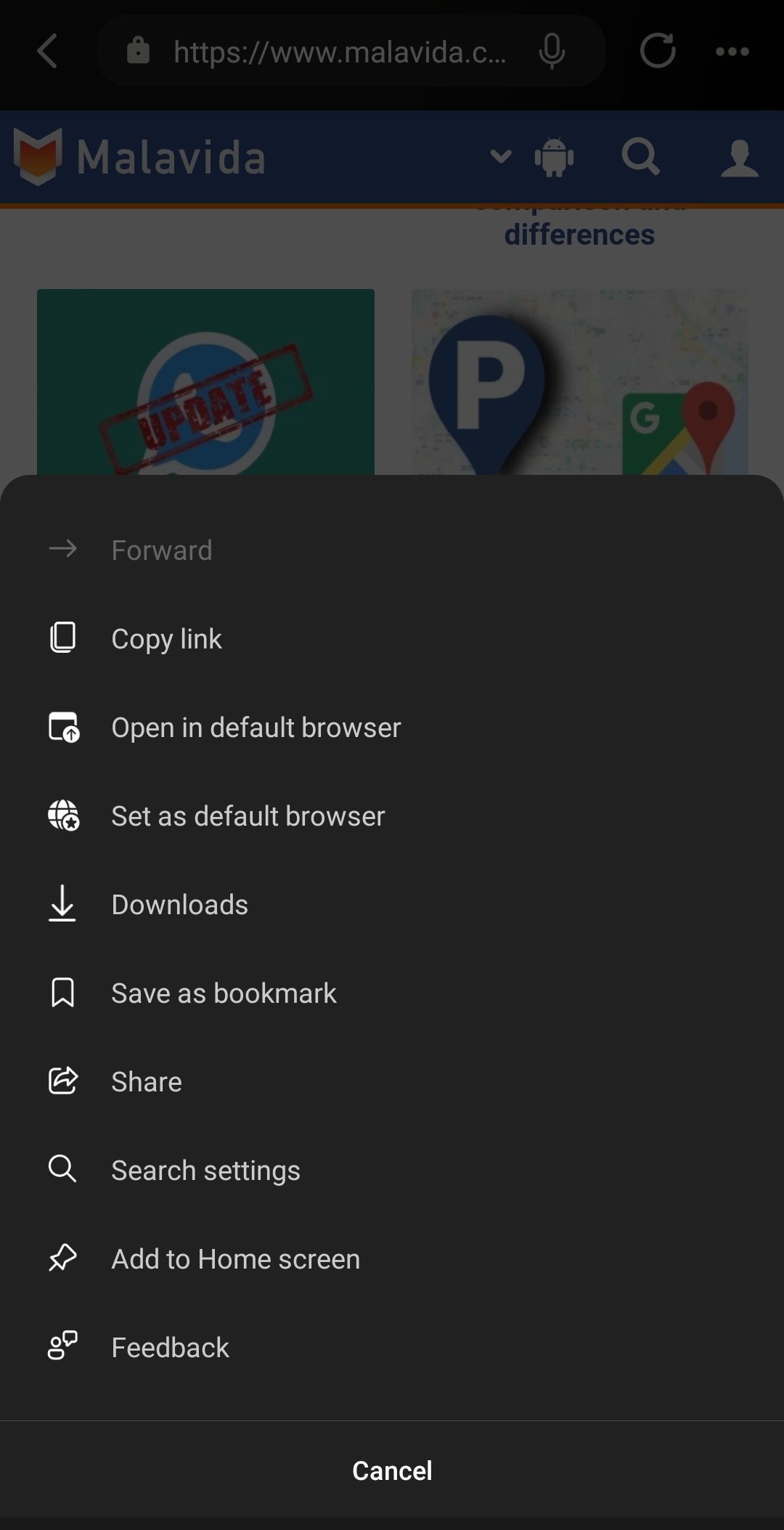The image depicts a screenshot taken from a cell phone, showcasing a webpage from the Malavida website, which is evident from the URL "https://www.malavida.com" displayed in the address bar at the top. The user interface includes a primarily black background. In the upper left corner, there is an arrow pointing to the left. 

The banner section of the website displays the Malavida logo, which consists of an orange and white design to the left of the word "Malavida" written in white text. On the upper right corner of the banner, icons for a white magnifying glass (representing search) and a profile image are visible. 

Below this banner, there is a green box featuring a blue and white circle that contains the image of a white cell phone. Superimposed on this circle is the word "update" in white. To the right of this box is a small section showing a Google Map. 

The remainder of the image is dominated by a list of options set against a black background, with white text. The list reads from top to bottom: 
1. Link
2. Open in Default Browser
3. Set as Default Browser
4. Downloads
5. Save as Bookmark
6. Share
7. Search Settings
8. Add to Home Screen
9. Feedback